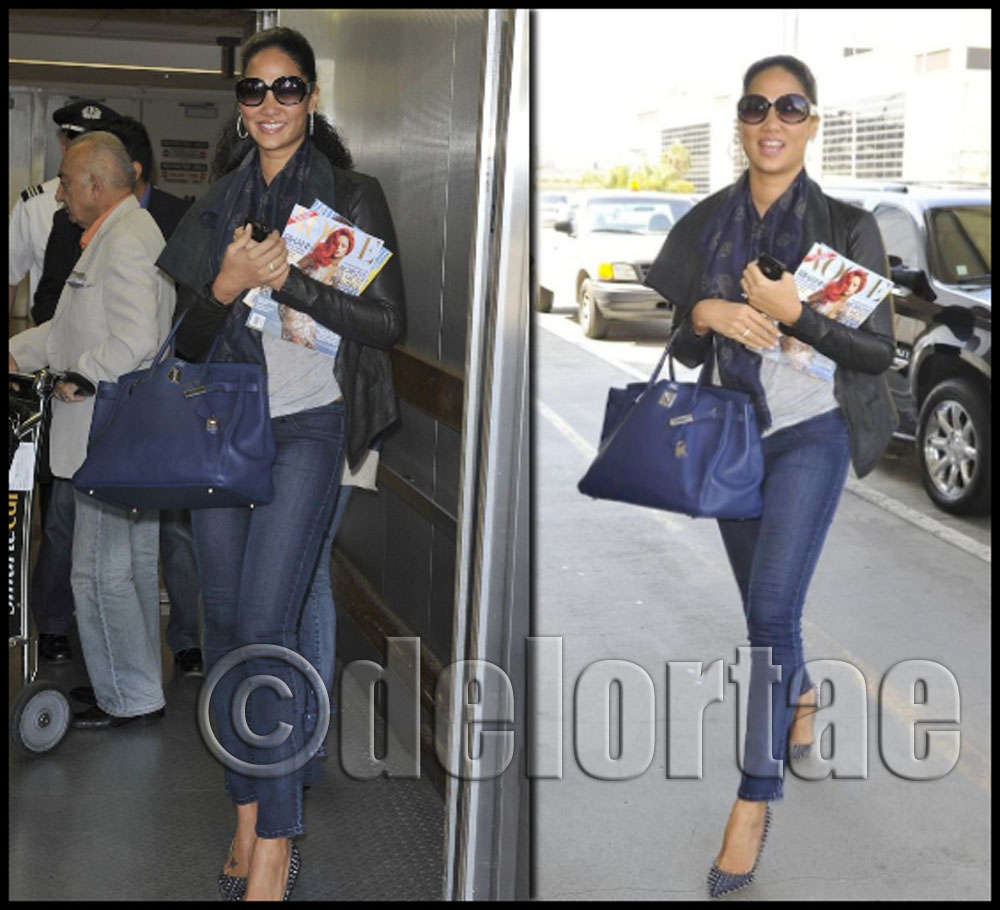The image consists of two side-by-side photographs featuring Kimora Lee Simmons. In both images, she is dressed identically in a black leather jacket over a gray shirt, complemented by a blue scarf, blue jeans, and high-heeled shoes with gem embellishments. Kimora's long, dark hair is pulled back, and she accessorizes with large, round sunglasses and hoop earrings. She carries a blue purse and several magazines in her left arm.

In the left photograph, Kimora is situated indoors, possibly in an airport elevator, with a flight attendant or pilot visible in the background. Several other people can also be seen, one of whom is pushing a cart. The right photograph shows Kimora on a sidewalk, with buildings and cars in the background, indicating she is now outside. Both images have the semi-transparent watermark reading "Copyright Delorte" across the bottom.